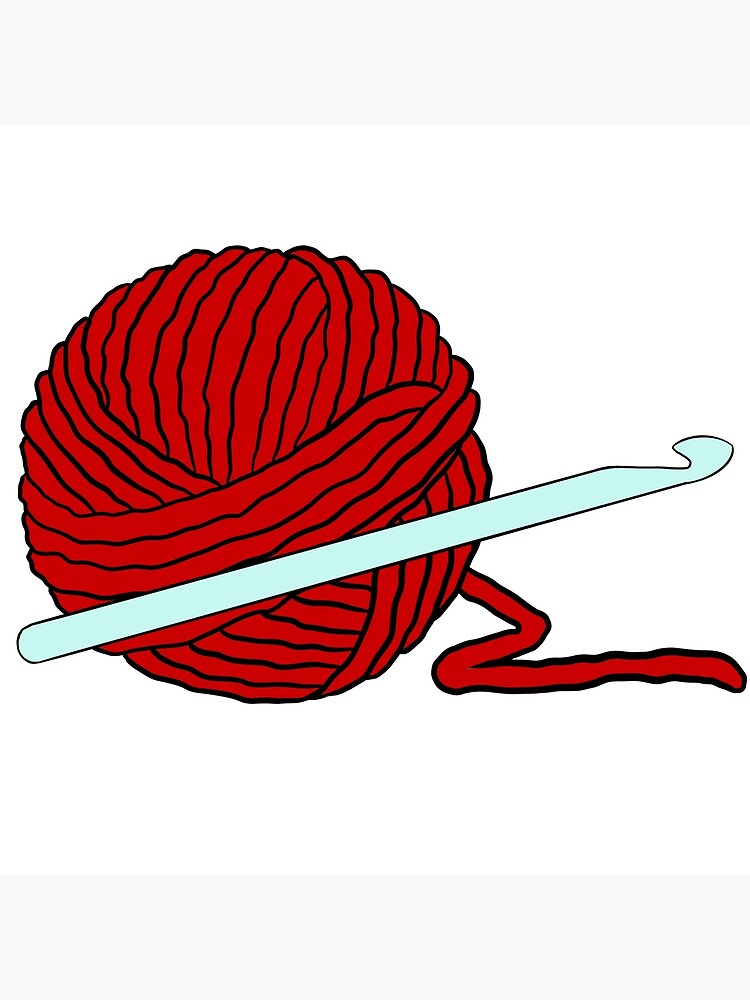This image is a detailed artist rendering of a medium-sized red ball of yarn and a short silver crochet hook, set against a white background. The ball of yarn, tightly wound with its string extending to the right, is drawn primarily with dark red and black ink, giving it a textured, typical appearance. The silver crochet hook, outlined in black and about four to five inches long, lies diagonally in front of the yarn, creating a visual contrast. The background subtly varies in shade, adding depth to the simple, floating composition where the hook appears almost suspended in midair.